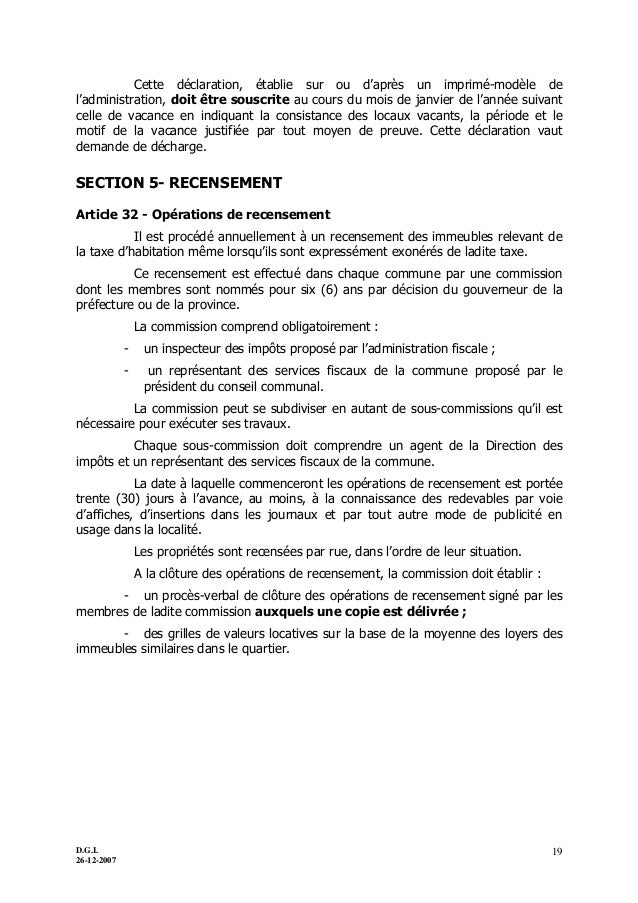The image is a cropped photograph of page 19 from a book. The page features a vertical rectangular layout with no borders, displaying black text on a white background. It is predominantly written in a language other than English. At the top, a small paragraph of text is followed by bold letters spelling "Section 5" and the word "Recensement." Additionally, it mentions "article 32" below this section. The page contains four bullet points and several paragraphs of regular and bolded text. In the lower right-hand corner, the page number 19 is visible, while the lower left-hand corner includes the notation "DGL 26-12-2007," indicating the date, December 26, 2007. Some very small writing is present in the far bottom corner.